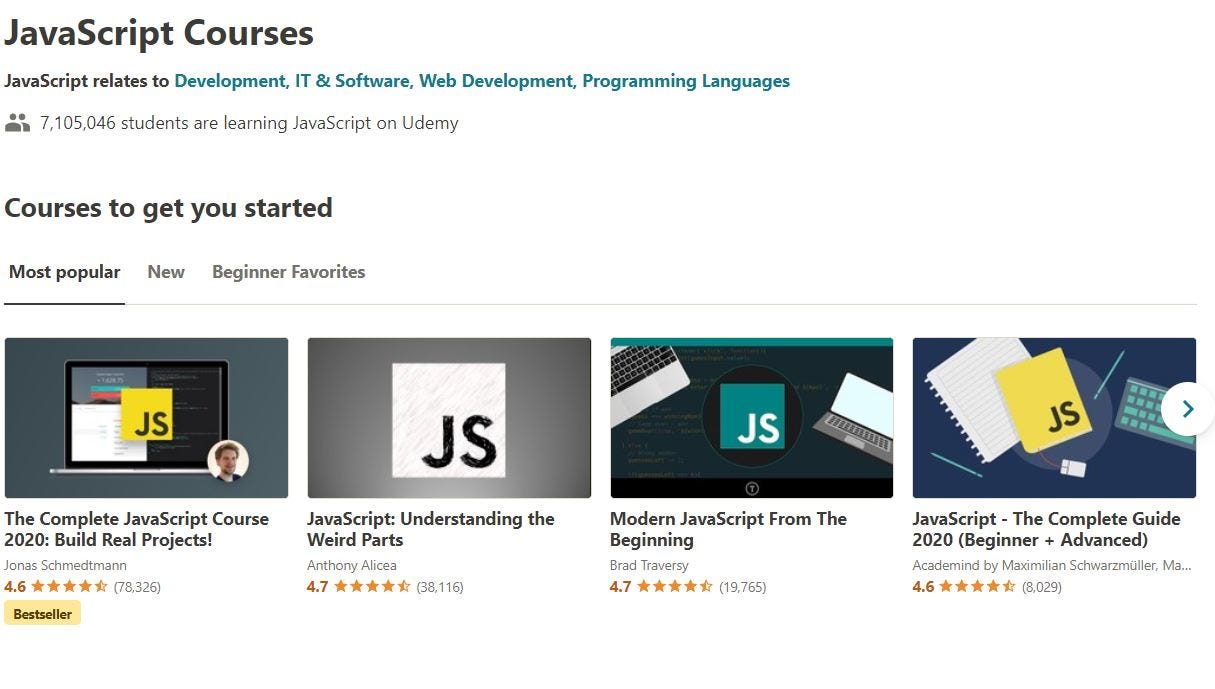**Detailed Caption:**

This image captures a portion of a Udemy webpage dedicated to JavaScript courses. The background is predominantly white, and at the top-left corner, there is bold black text that reads "JavaScript Courses." Just below this heading, in smaller text, it reads: "JavaScript related to..." followed by green-colored categories including "development," "IT & software," "web development," and "programming languages."

Further down, there's an icon depicting two people, with a caption stating "7,105,046 students are learning JavaScript on Udemy." Following this, there is another black text heading that declares "Courses to get you started." Below this heading are three tabs: "Most Popular," "New," and "Beginner Favorites." The "Most Popular" tab stands out in bold black text, while the other two tabs are grayed out.

Towards the bottom of the webpage, there are four rectangular thumbnails, each representing a different JavaScript course. These thumbnails feature various graphical elements such as "JS" letters overlaid on laptops, a white and gray background, a circular icon with a green square, and laptops positioned beside or on top of notebooks. Below each thumbnail, there is a title in black text along with user ratings out of five stars. From left to right, the course details are as follows:

1. **The Complete JavaScript Course 2020 Build Real Projects**: Rated 4.6 stars based on 78,326 reviews. This course features a yellow rectangle at the bottom-left corner with black text, "Bestseller."
2. **JavaScript Understanding the Weird Parts, Anthony Alessia**: Rated 4.7 stars from 38,116 reviews.
3. **Modern JavaScript From the Beginning**: Rated 4.7 stars from 19,765 reviews.
4. **JavaScript, the Complete Guide 2020 Beginner to Advanced**: Rated 4.6 stars from 8,029 reviews.

This webpage layout and detailed options offer a comprehensive overview of available JavaScript courses for users interested in learning or enhancing their skills through Udemy.